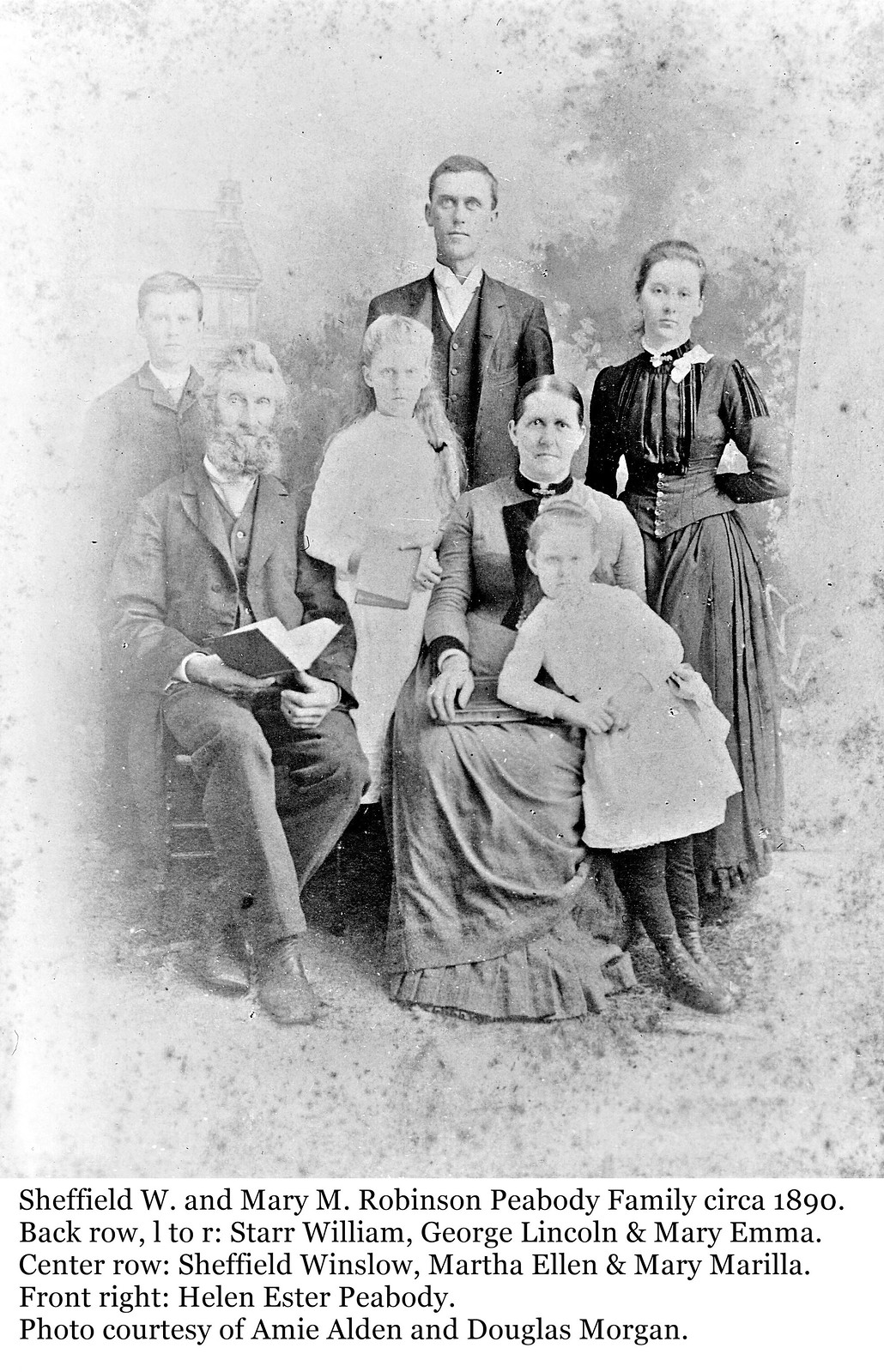This is a vintage black-and-white family photograph from circa 1890, featuring seven individuals. In the back row, from left to right, stand two adult men and one adult woman identified as Star William, George Lincoln, and Mary Emma. In the center row, an elderly man with a beard, named Sheffield Winslow, is seated and holding a book, with a young girl, Martha Ellen, standing next to him. Seated in the front row is an adult woman, Mary Marilla, with a young girl, Helen Esther Peabody, standing in front of her. The individuals are dressed in period clothing: the men in black suits, the women in long dresses, and the young girls in long white dresses. No one in the photograph is smiling. The photo also has a backdrop that partially reveals a house. The text below the image reads, "Sheffield W. and Mary M. Robinson Peabody Family, circa 1890. Back row left to right: Star William, George Lincoln, and Mary Emma. Center row: Sheffield Winslow, Martha Ellen, and Mary Marilla. Front row: Helen Esther Peabody. Photo courtesy of Amie Alden and Douglas Morgan."